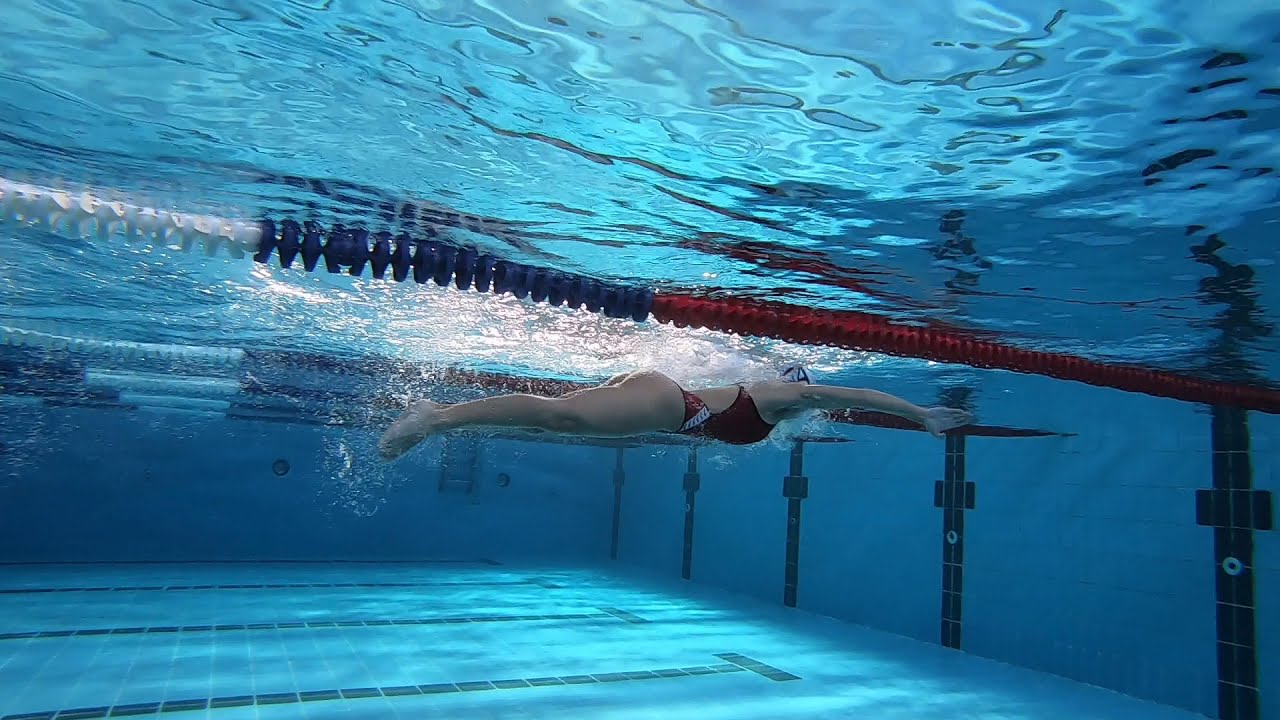This is an underwater photograph taken in an indoor, Olympic-type swimming pool with distinct lanes for swimming laps. At the bottom of each lane, there is a T-shaped black line, and vertically oriented black lines mark the side boundaries. A red, white, and blue rope runs along the length of each lane, indicating the lanes' borders. The image captures a muscular woman in a red bathing suit, swimming toward the end of her lap. She wears a blue and white bathing cap and is in mid-stroke, with her arms extended out to the sides and her face not visible as it’s immersed in the water. Her body is outstretched, and she kicks her feet behind her. The water above her is visibly disturbed with a white splash, reflecting her movements. The pool's blue tiles and various black lane markings are clearly visible underwater, contributing to the geometric precision of the scene.